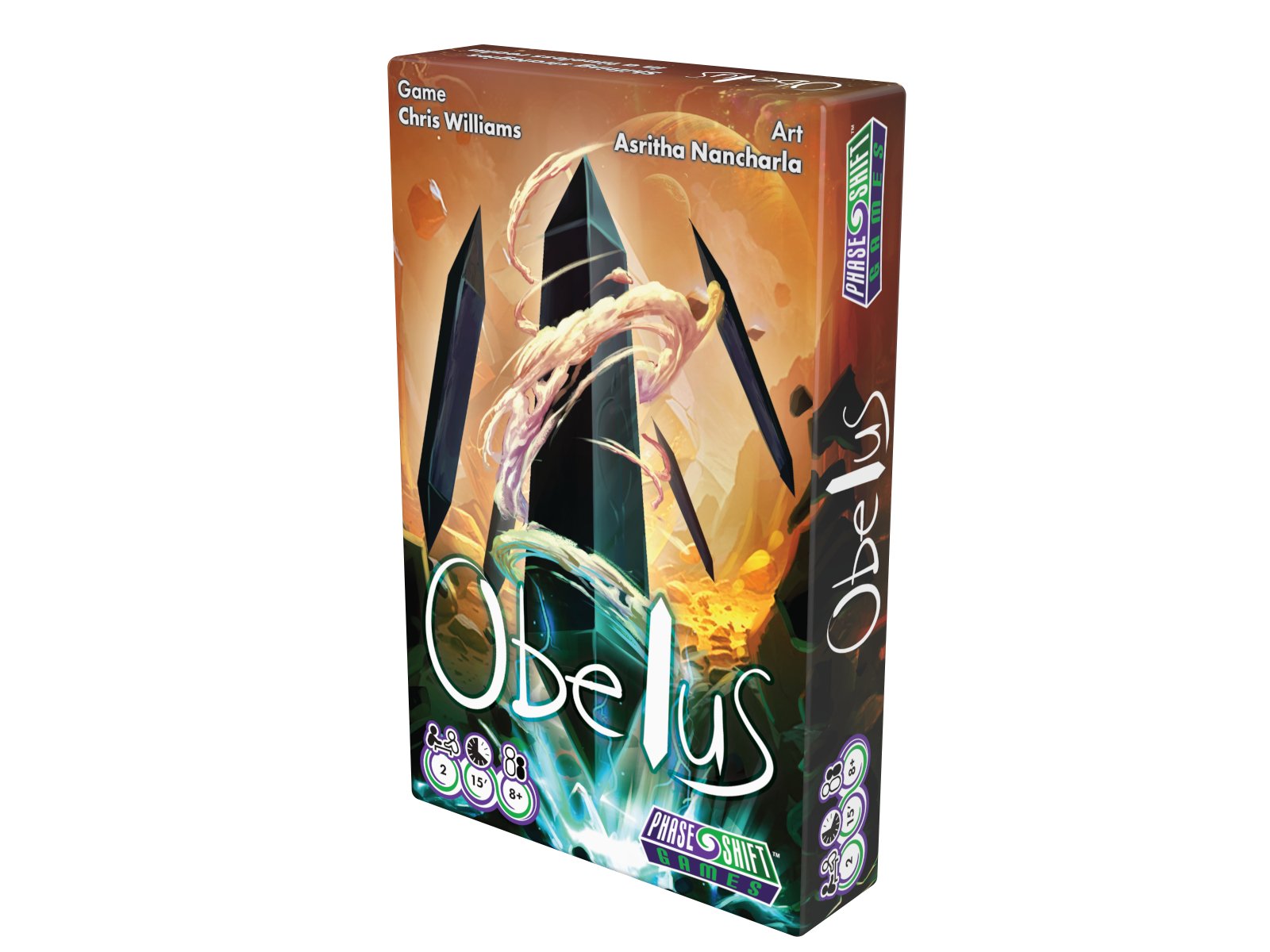The image showcases a striking board game box, set against a solid white background that dominates the composition. The box itself is predominantly brown and orange, with complex illustrations adorning its front cover. These illustrations include black floating stones with pyramid-shaped tops and bottoms, surrounded by mystical clouds and set against an orange sky featuring planets. The front cover prominently displays several text elements: in the upper left corner, it says "Game, Chris Williams," while the upper right corner reads "Art, Azritha, Nancharla." The bottom of the box bears the title "Obelis" and in the lower left corner, the publisher "Phase Shift Games." The side face of the box is also partially visible, adding depth to the scene and emphasizing the game's intricate design and artistic elements.